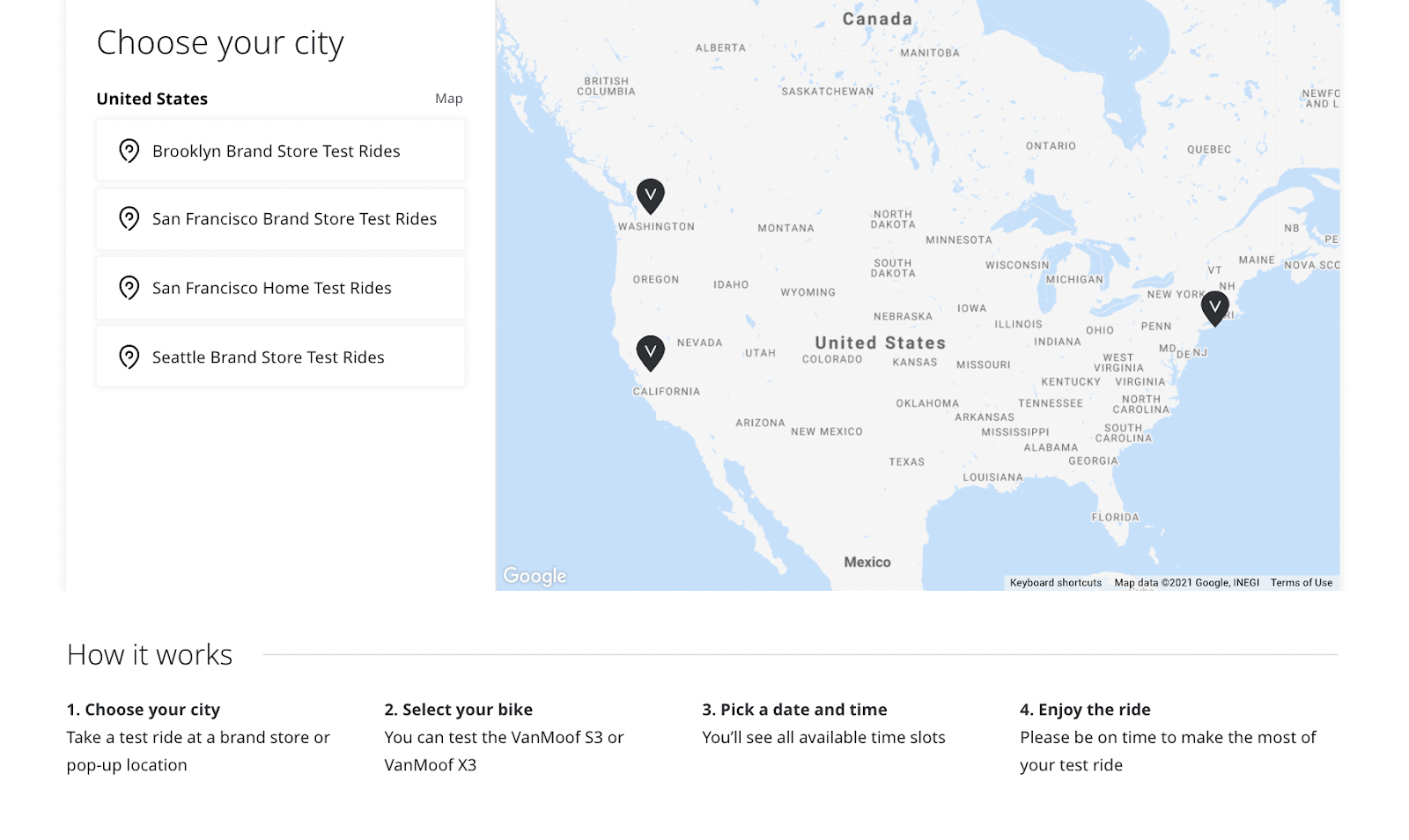This detailed caption describes an informative map of North America highlighting test ride locations for VanMoof bikes in the United States. At the top, you can see Canada, followed by the United States, and Mexico at the bottom. The map features pointers with a distinct black design marked with a white "V", indicating test ride centers. Notable locations pinpointed include Seattle in Washington State, San Francisco in California, and Washington, D.C., on the East Coast.

The map invites users to "Choose Your City" to participate in test rides at various VanMoof brand stores and public locations. Specific options include test rides at the Brooklyn brand store, San Francisco brand store, and home test rides in San Francisco, as well as the Seattle brand store.

A step-by-step guide on how the process works is included:
1. Select your city.
2. Choose a test ride location at a brand store or public venue.
3. Pick your bike model, either the VanMoof 53 or the VanMoof X3.
4. Schedule your ride by selecting an available time slot.
5. Enjoy your test ride, ensuring timely arrival for the best experience.

Although the map does not feature a logo or images of the bikes, it provides comprehensive instructions for enthusiasts interested in testing out VanMoof bicycles.